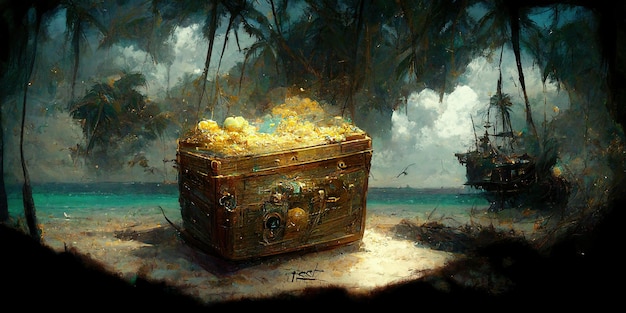The painting is a detailed depiction of a treasure chest scene on a beach, measuring approximately four to five inches in width and two to three inches in height. At the center of the composition, a lidless wooden treasure chest overflows with gold baubles and coins, some spilling out onto the sand. The chest is brown with bronze accents or support braces, and appears to have some undetailed jeweled embellishments on its front.

Surrounding the chest is a sandy area, framed by a border with dark vignetting and brown edging, partially obscuring the foliage around it. Overhead, low-lying leaves and branches from nearby trees dangle, integrating into the scene. Behind the chest, the turquoise ocean stretches into the distance, where an old pirate ship is visible, either docked or sailing away, on the right-hand side. The scene is further accentuated by a turbulent sky filled with white and gray clouds, suggesting an approaching storm. Above the horizon, birds can be seen flying, adding a sense of motion to this intricate seaside tableau. At the bottom of the image, the artist's signature is present, marking the piece with authenticity.